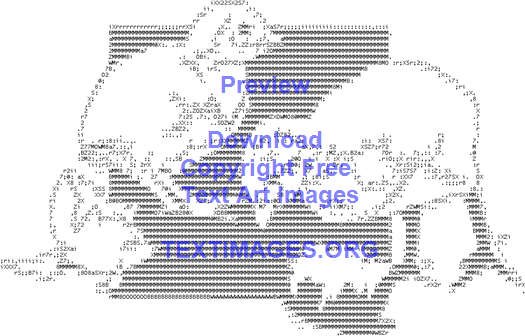This detailed caption describes a digital artwork created using letters and numbers reminiscent of old-school dot matrix printers. The image depicts two baby chicks, each emerging from a half-cracked eggshell. The chick on the left has white legs and stands beside a white eggshell, while the chick on the right has black legs and a black bottom shell. The right chick appears to be pecking for food. The main part of the image is set against a black square on a light gray background. Above the artwork, in purplish-blue text, it reads "Preview" followed by "Download copyright-free text art images" and "textimages.org." The text was made bold to form the black portions of the image, contributing to the overall black-and-white aesthetic.